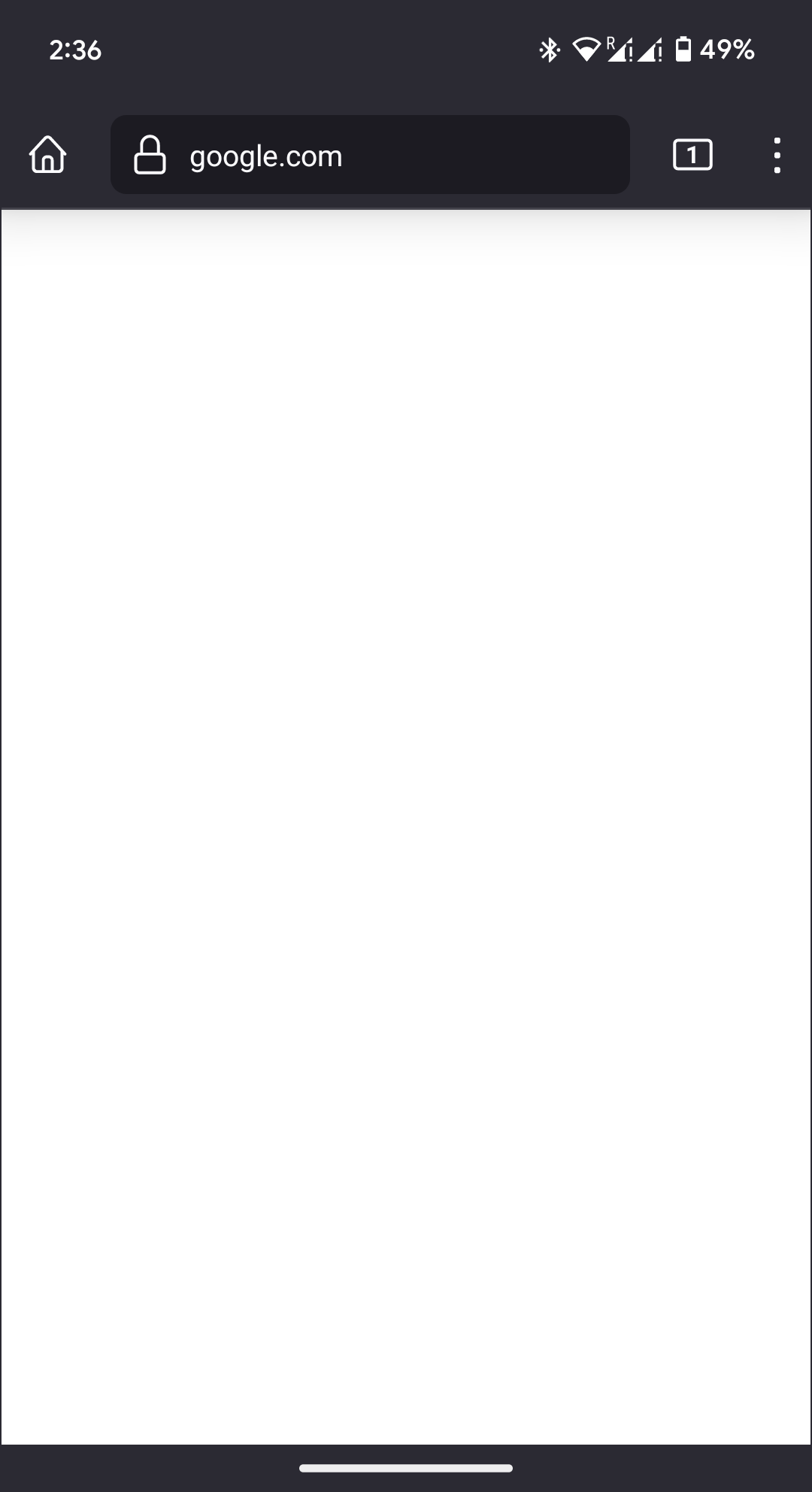In this screenshot captured from an unidentified mobile device, the user interface displays several typical mobile elements. The status bar at the top shows it is 2:36 PM, and provides various icons: a Bluetooth symbol, a Wi-Fi symbol, two data symbols marked with an error exclamation point, and a battery indicator showing 49% charge in a half-filled icon.

The main screen is of a browser or possibly the Google app, where the user is attempting to access google.com. However, the webpage is entirely blank, suggesting a loading issue or an incomplete capture. The URL "google.com" is visible in the address bar, accompanied on the left by a lock symbol indicating a secure connection, and a home icon even further left. On the right of the URL, there is a tab indicator showing the number "1", signifying that only one tab is currently open, next to three vertical dots which typically open further browser options.

The color scheme of the interface is primarily dark gray and white, matching common design aesthetics for readability and simplicity. The blank page likely implies either a connectivity issue or a premature screenshot before the page loaded fully.